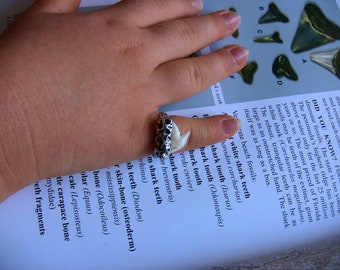This indoor photograph captures a close-up view of a book page displaying various labeled images of shark teeth, such as those of a great white shark, accompanied by corresponding text descriptions on the left or toward the bottom. The focal point of the image, however, is a woman's right hand resting on the page, obscuring parts of the shark teeth pictures. The hand is somewhat chubby with long, unpainted nails, and lacks definition at the knuckles. Covering her pinky finger is a distinctive sterling silver ring featuring a textured, porous surface with black divots and a white shark tooth mounted on top. The top of her hand, including her thumb, is out of the frame, leaving only her four fingers visible as they cover another photograph beneath the shark teeth images. The background of the book page is white with contrasting black text.